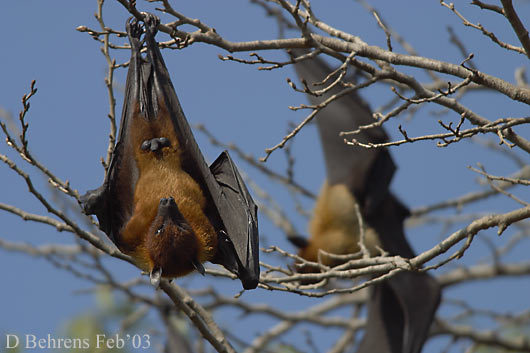Against a light blue sky, tree branches stretch out without any buds or leaves. Hanging upside down from the branches are two bats. The closest bat, which is clearly visible, has a brown body and a darker brown face. Its wings are folded tightly against its body, and its chin appears tucked to its chest. The bat has little pointy ears and clings to the branch with its legs. Its wings are dark gray and appear super thin. In the background, the second bat is more blurred, with its wings seemingly extended. Both bats exhibit the characteristic bat anatomy with black wings and feet. At the bottom left corner of the image, there is faint white text in Times New Roman that reads "D. Behrens Feb '03."